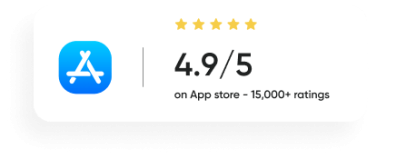The image features a small graphic prominently displaying the App Store logo, characterized by three white popsicle sticks arranged to form the letter "A" against a blue square with rounded edges. Adjacent to the logo is a rating section, showcasing five illuminated stars and a near-perfect rating of 4.9 out of 5. Beneath this rating, the text reads "on App Store - 15,000+ ratings." The image appears to be designed for showcasing the high rating of an unspecified app on the Apple App Store.